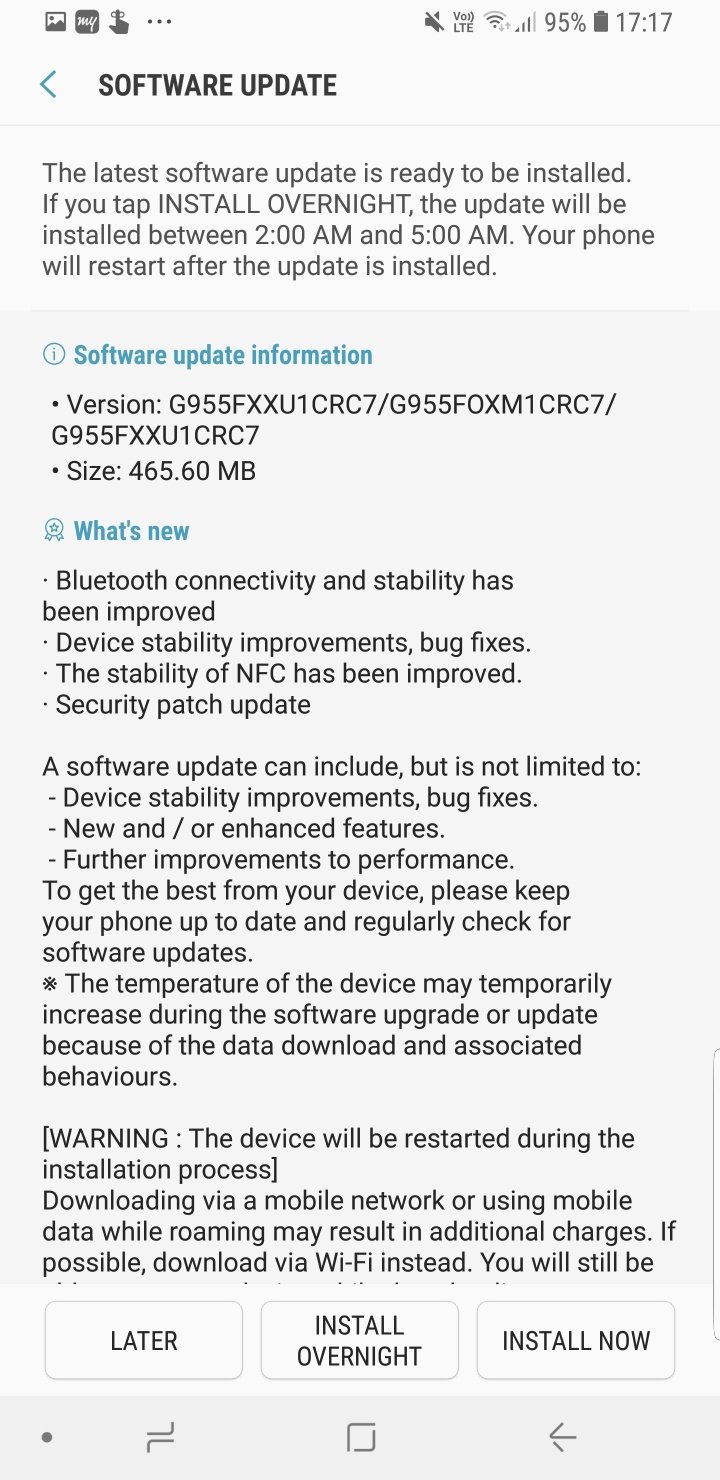This is a detailed screenshot of a software update page on a smartphone. 

At the very top of the screen, there is an icon bar displaying various notifications and indicators. From left to right, there is a picture icon, an unidentified icon, and a hand icon that appears to be pointing at something, followed by three dots representing additional options. On the far right, there is a volume-off icon and several service indicators, including LTE, Wi-Fi, signal bars, and a battery icon showing 95% charge. The time is displayed as 17:17.

Below the icon bar, the title bar of the page reads "Software Update" in black text. On the left side of this bar, there is a blue back button. Underneath the title bar, there is a brief message in black text stating, "The latest software update is ready to be installed. If you tap 'Install overnight,' the update will be installed between 2 a.m. and 5 a.m. Your phone will restart after the update is installed."

Following this message, there is a gray box containing more detailed information. At the top of this box, "Software Update Information" is written in blue text alongside an information icon. Beneath this, the version and size of the update are listed in black text. Further down, there is a section titled "What's New" in blue text, accompanied by an award icon, detailing the new features and improvements in black text.

At the bottom of the gray box, there are three white buttons with gray outlines. The buttons are labeled "Later," "Install Overnight," and "Install Now." Finally, at the very bottom of the screen, there is a navigation bar with three buttons: a recent apps (tabs) button, a home button, and a back button.